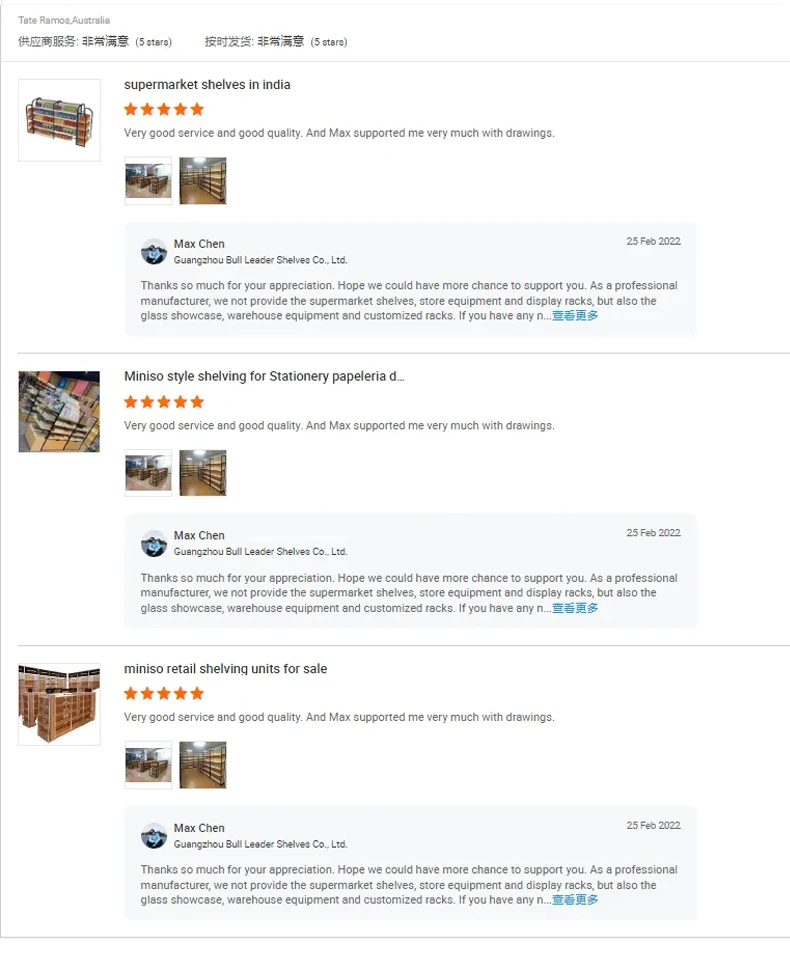The image displays a website interface with a clean, white background and a layout featuring three detailed customer reviews. 

**Header:**
In the upper left corner, "Tate Ramos Australia" is prominently displayed, succeeded by Chinese text. Within parentheses next to the Chinese text, "five stars" is written, indicating high reviews. 

**First Review:**
The top review features a small square image of supermarket shelves in India on the left. The accompanying text reads: "Supermarket shelves in India. Five orange stars. Very good service and quality. Max supported me a lot with drawings." There are two additional smaller pictures of shelves below the main image. 
- A light gray rectangle follows, containing the text: "Max - 10, Guangzhou Bull Leader Shelves Company Limited. Thank you so much for your appreciation. We hope to have more opportunities to support you. As a professional manufacturer, we not only provide supermarket shelves, store equipment, and display racks but also glass showcases, warehouse equipment, and customized racks. If you have any..." ending with an ellipsis. 
- A clickable blue Chinese character, likely indicating "read more," is located at the end. 
- The date "25 Feb 2022" is visible at the top right of the gray rectangle.

**Second Review:**
The second review mirrors the first in formatting. A square image of a "Mini Sol-style shelving for stationary" is positioned on the top left. The text reads: "Five orange stars. Very good service and quality. Max supported me a lot with the drawings." Two smaller pictures of shelves follow.
- An identical light gray rectangle with the same manufacturer’s thank-you message is below. 
- The same clickable blue Chinese character appears at the end. 
- Date: "25 February 2022."

**Third Review:**
The third review follows the same format but with a different headline and slight textual adjustments. The headline reads: "Mini cell retail shelving units for sale. Five stars. Very good service and quality. Max supported me with everything." 
- The initial picture of shelves in this review is distinct from the previous two.
- It includes the same two smaller images and the identical gray rectangle with the manufacturer's thank-you message.
- The date is again "25 Feb 2022."

Throughout the image, each section is separated by thin, light gray lines, maintaining a neat and organized appearance.